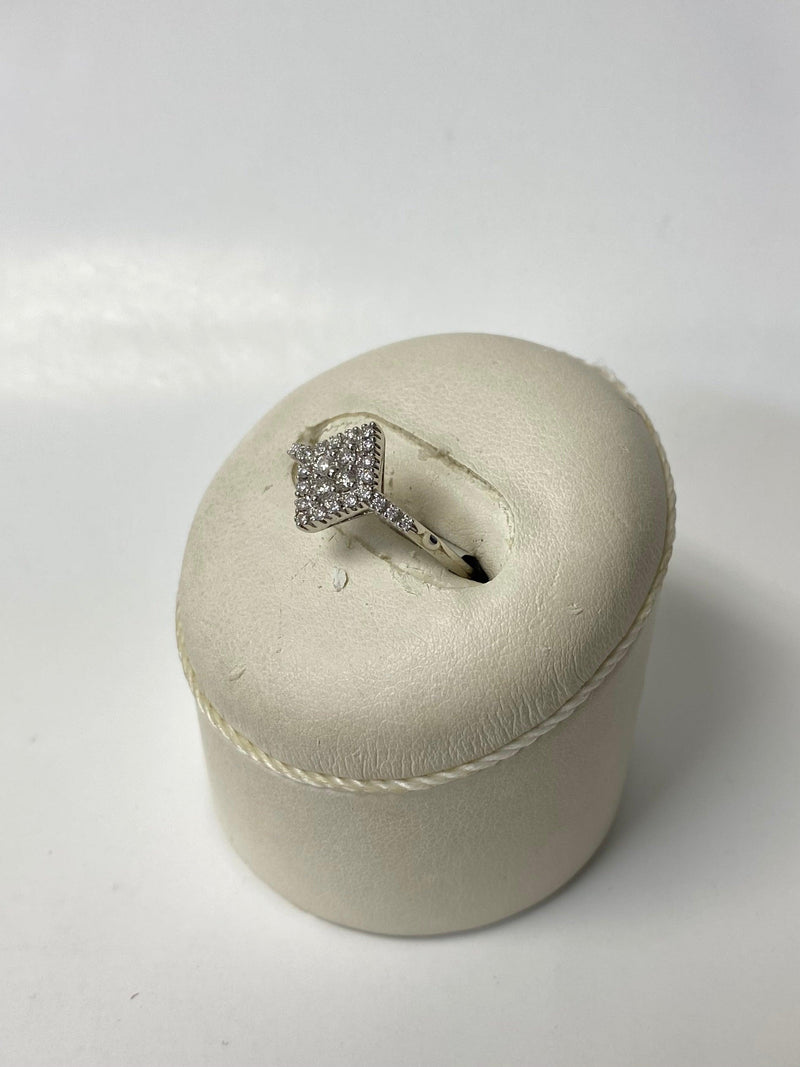This photograph showcases a stunning silver ring, polished to perfection and adorned with an array of sparkling diamonds. The ring, which features a square-shaped top densely encrusted with larger diamonds in the center and smaller ones around the edges, rests on a soft, beige podium typical of elegant jewelry displays found in diamond stores. This podium, resembling a plush pillow, is slightly tilted to enhance the viewing angles of the ring, allowing the diamonds to catch the light beautifully. The soft holder, which includes a delicate string embellishment around its circular base, presents the ring prominently and securely. This entire setup is situated against a clean, white background, ensuring all attention is drawn to the exquisite details of the ring and its luxurious display.